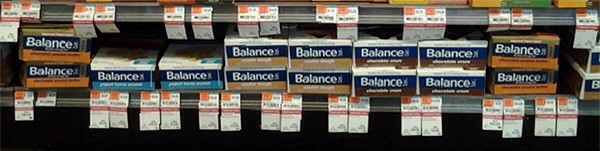This image showcases a section of grocery store shelves, specifically displaying various brands of a product named "Balance." The shelves feature four distinct versions of this product, each differentiated by color-coded designs and likely price tags hanging from the shelves indicating potential savings.

On the extreme left, the "Balance" product is distinguished by a striking dark black background with 'Balance' written in white text. Beneath the white text, there's an orange stripe. Mirroring this on the far right side is a similar product design, also featuring the same black background and orange stripe.

Adjacent to the far-left package, the next "Balance" product also maintains a dark background, though this one leans more towards navy blue. Below the branding, a light blue stripe adds contrast to the packaging. Next in line, the subsequent "Balance" product keeps the navy background, but adds a golden stripe beneath the brand name, giving it a more premium feel. Finally, the last "Balance" product shown has a black cherry red stripe underneath the 'Balance' branding, making for a bold and eye-catching design.

Each of these designs is aligned in two rows, clearly organized to offer a variety of options to customers shopping for "Balance" products in this grocery store.